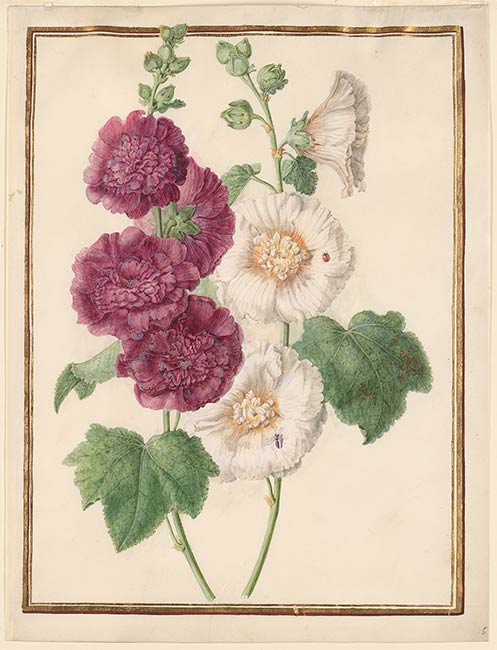This image is a detailed painting of two flowering plants on a cream background. It is set within a double-lined gold border, creating a rectangle shape in portrait layout, meaning the height is greater than the width. The left side features a vertical stem with four maroon, multi-petaled flowers and vibrant green leaves. The right side showcases a vertical stem with three white, multi-petaled flowers accented by a yellow center, also surrounded by green leaves. Notably, a few small insects are visible on the white flowers. The detailed artwork highlights the intricate elements of each petal and leaf, rendering the overall depiction quite ornate and vivid.